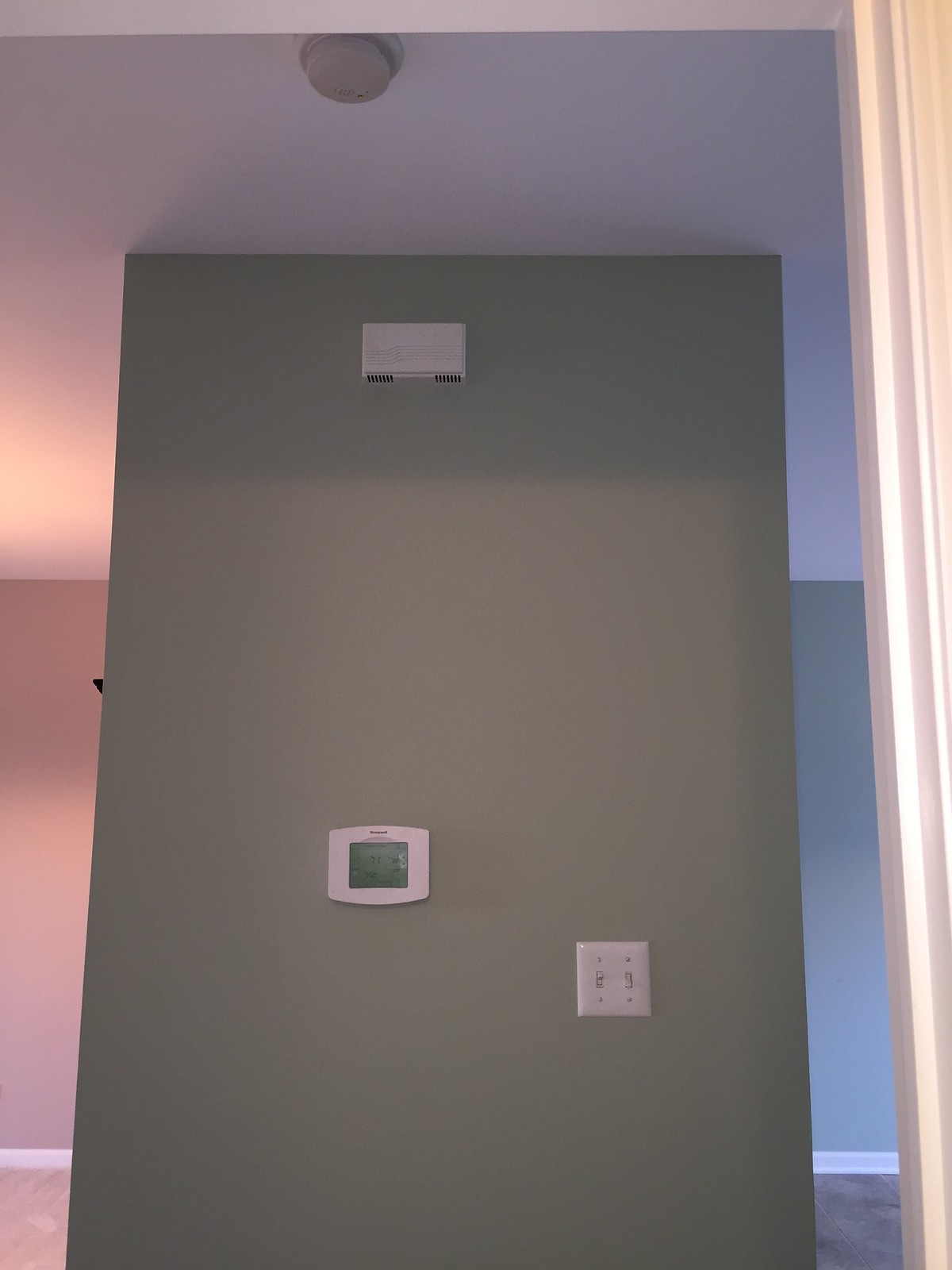This photograph captures the interior of a house, showcasing various elements with rich detail. Dominating the upper section, the white ceiling extends uniformly, interrupted only by a suspended circular light fixture. Below, a green wall meets the ceiling seamlessly, onto which a white air conditioning unit is mounted, identifiable by its sleek, rectangular shape. Just beneath the air conditioning unit, a second device with a screen—white in casing with a green display—adds to the wall's functional decor. Amidst these, a cable cord and a switch are conspicuously attached, providing a sense of utility.

The background further diversifies the color palette: a prominent blue wall rises on the right, showing subtle gradients of white and gray towards its base, enriching its texture. Intersecting this, a pink wall emerges, adding a vibrant contrast on the far right. Grounding the scene, a white baseboard runs along the bottom, delineating the transition between wall and floor while enhancing the room's architectural detailing.